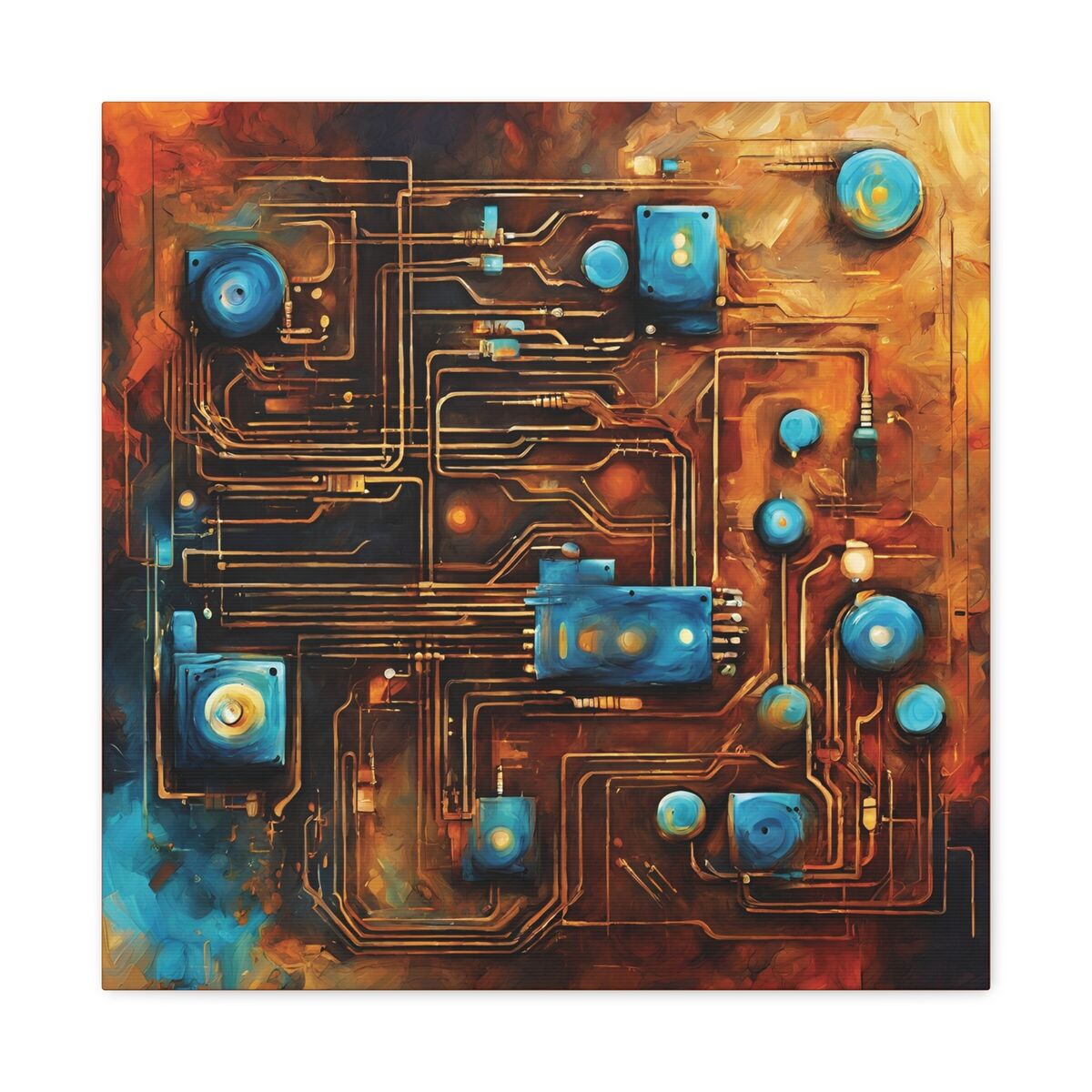This image depicts an abstract, modern art interpretation of an electronic circuit board, rendered in the style of a detailed drawing. The background features a swirling palette of amber, orange, and brown hues, with hints of greenish blue in the bottom corner, giving it a steampunk-like atmosphere. A network of meticulously painted yellow wires crisscrosses the board in a grid-like pattern, connecting various electronic components that are geometrically arranged.

Dominating the scene, a bronze-colored metal base hosts a diversity of chips and parts. From left to right, a round chip appears first, followed by a grid work of yellow-colored wires leading to a blue rectangular chip. Adjacent to this are two yellow dots and another small yellow dot chip. The top right-hand corner presents a blue round chip with a yellow dot at its center.

In the bottom right-hand corner, three blue chips, some adorned with white dots and one with a yellow dot, come into view, alongside a rectangular chip. Centermost is a prominent blue rectangular chip accented with red, yellow, and white buttons. The lower portion includes a rectangular chip with a yellow button in the bottom left-hand corner and a blue square chip featuring a yellow dot in the middle. Scattered red dots accentuate the midsection, enhancing the artwork’s complexity.

The entire composition, encased within a square frame, vividly illustrates a creative, almost whimsical reimagining of a circuit board, where wiring mimics a street map and components take on artistic liberties, blending functionality with imaginative abstraction.